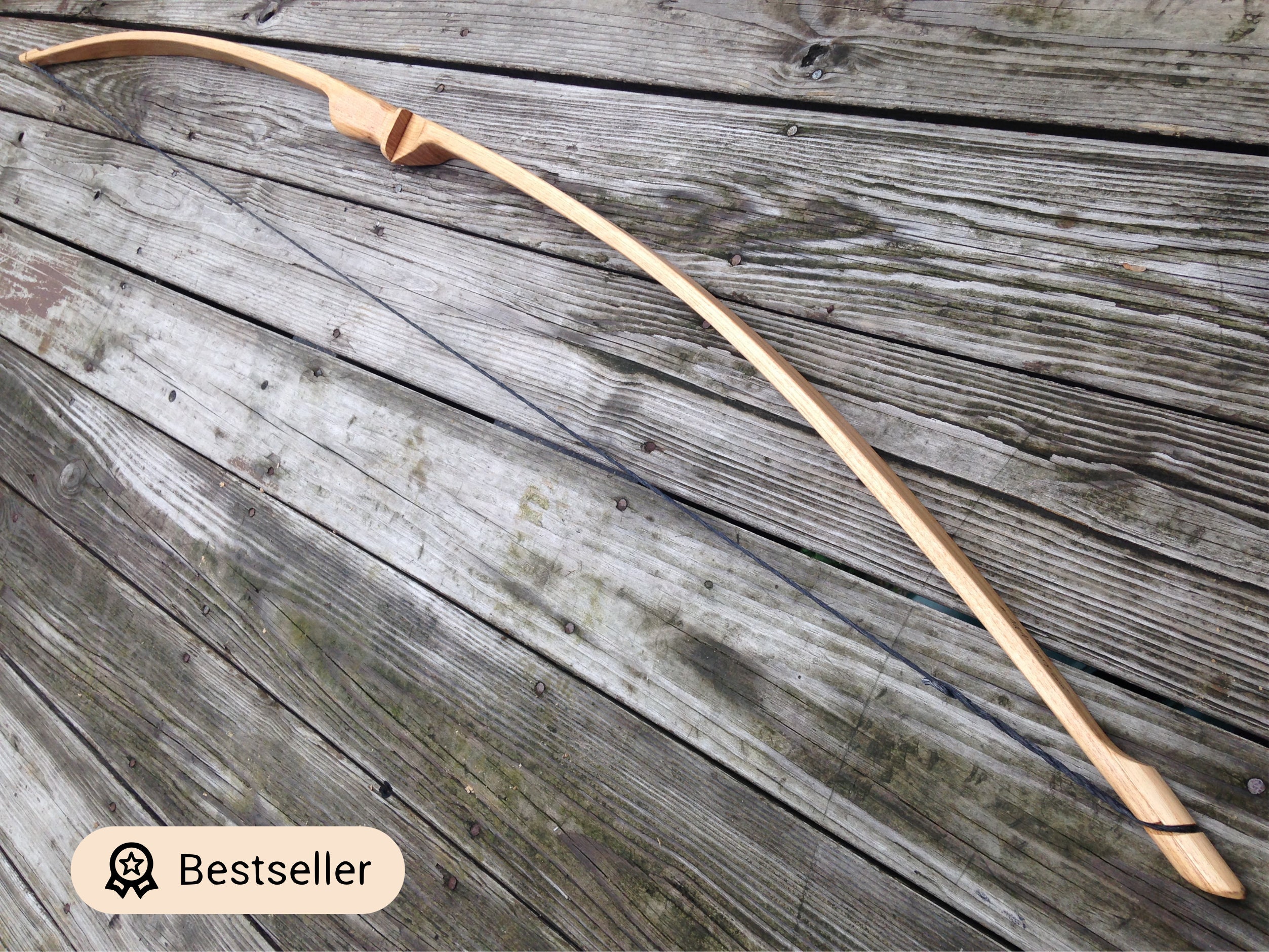This image captures a detailed scene of a handmade bow, likely listed for sale on Etsy.com, indicated by an overlay watermark reading "Best Seller" in distinct black text with a ribbon on a light off-white oval in the bottom left corner. The bow, crafted from beige-colored wood, is positioned sideways on an aged wooden deck, which contrasts starkly with the bow due to its gray, weathered appearance. The deck's planks show signs of deterioration, including white and gray areas, and patches of green mold. The bow itself curves gracefully from the bottom right to the top left of the image, featuring a single dark blue string. In the middle of the bow, there is a clear notch or crease designed to hold an arrow. The setting is illuminated by natural daylight, which helps to highlight the bow's craftsmanship and the textured details of the surrounding wooden surface.